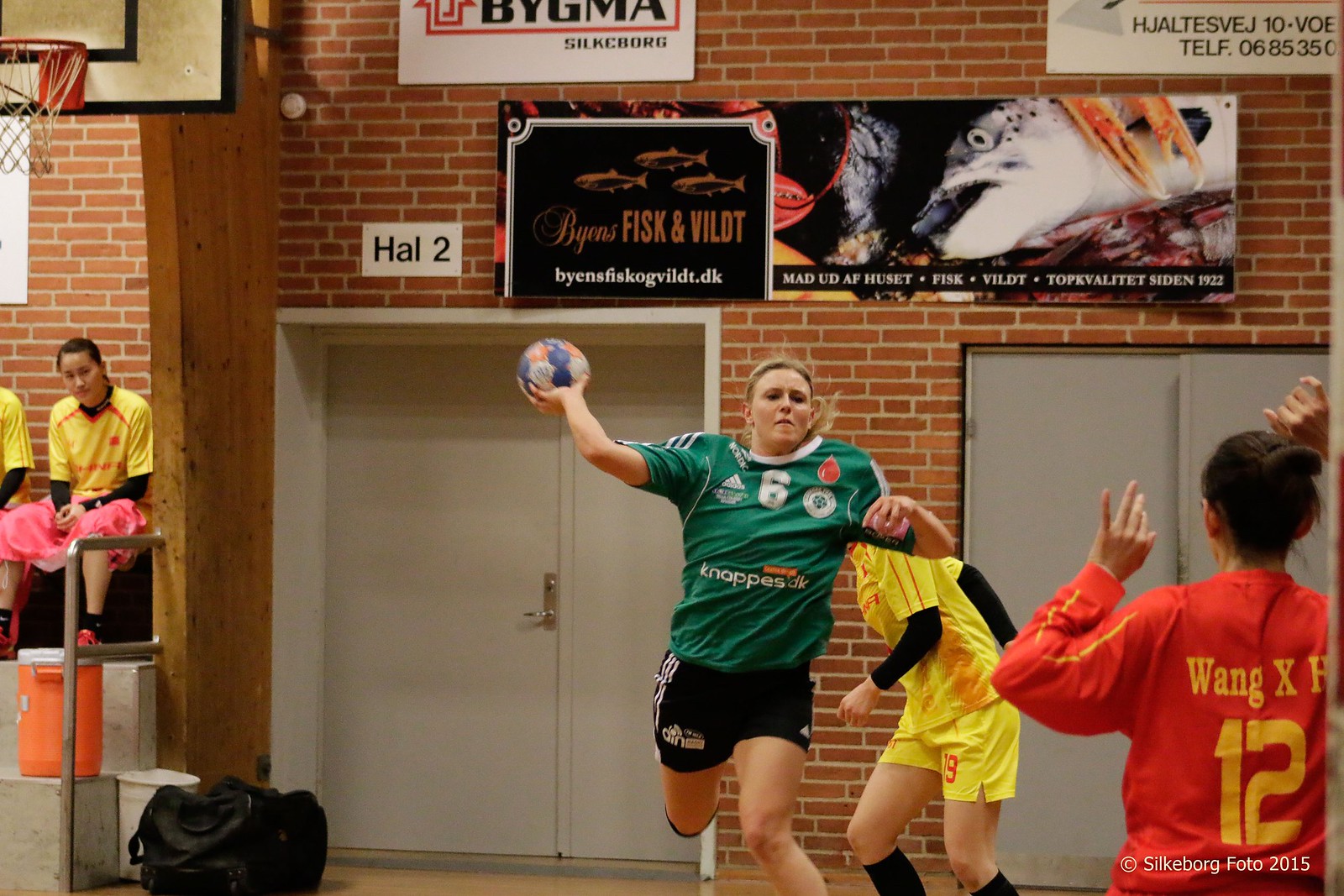The image captures an indoor gymnasium with brick-patterned walls adorned with various banners and posters. The scene depicts an intense game involving three female players on the court. A white, blonde-haired player wearing a green jersey and black shorts holds a ball in her right hand, poised to throw it. Behind her stands another player in a yellow jersey and shorts. To the right, an athlete with "Wang X-12" on her red long-sleeve jersey has her back turned towards the camera, her black hair tied up, both arms raised. In the background, several spectators wearing yellow jerseys are seated in the stands. The gymnasium features double doors and a conspicuous basketball hoop on the upper left-hand side of the image. The court’s markings and the players' uniforms suggest this could be a hybrid sport resembling basketball but using a different type of ball. The image is watermarked "Silke Wong Photo 2015."